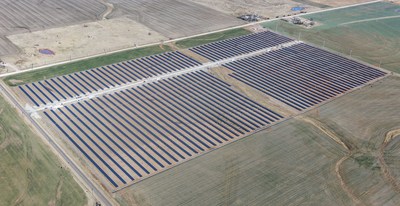The image captures an aerial view of a large, rectangular field in a desert-like area. The field is composed of rows of solar panels, distinguishable by their dark blue, purplish hue, which contrasts with the surrounding tan and slightly gray dirt. A prominent white line runs horizontally across the field, about three-quarters of the way up. The field is bordered by mildly green patches and flanked by a road, indicating some human activity amid the arid landscape. Despite the bright appearance, the sky is not visible in the daytime shot.